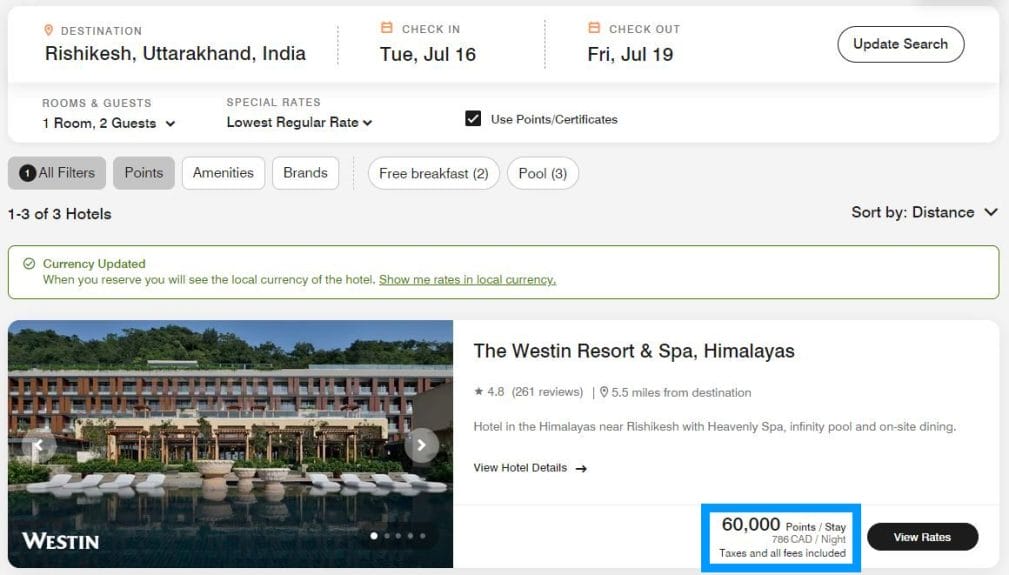This vibrant color image appears to be a snapshot of a travel website, specifically showcasing a hotel booking page for a destination in Rishikesh, Uttarakhand, India. In the top left corner, the destination is clearly marked: "Rishikesh, Uttarakhand, India." The user has selected travel dates with a check-in on Tuesday, July 16th, and a check-out on Friday, July 19th. The "Update Search" button is prominently positioned on the right-hand side.

Additionally, the details of the room and guests are indicated, with one room reserved for two guests. Special rates are highlighted, with the "Lowest Regular Rate" option checked off. There's a black tick box marked for "Use Points Certificates." Below this section, the filter options and point categories such as amenities and brands are marked in grey.

Highlighted is a promise of free breakfast and amenities like a pool. Specifically, the page notes "two pools" and "three amenities," with the number "three" displayed in white. Over "133 hotels" are listed, and sorting options by distance are available on the right-hand side.

A green text rectangle updates currency information: "When you reserve, you will see the local currency of the hotel," and offers an option to "Show rates in local currency".

Prominently featured on the right-hand side is an image of the hotel's exterior. The scenery includes a blue sky, some trees in the background, and water reflecting the surroundings in the foreground. The hotel's name, "The Western Resort, Hotel and Spa, Himalayas," is written in white on the lower left corner of the image, indicating a high rating of 4.8 stars based on 281 reviews, and located 5.3 miles from the destination. The description highlights amenities like a heavenly spa, infinity pool, and on-site dining.

A detailed view of the hotel reveals it costs 600,000 points for rewards members or a listed price of CAD 7,086 per night, inclusive of taxes and fees. At the extreme lower right, a "View Rate" button is visible, in black with white text.